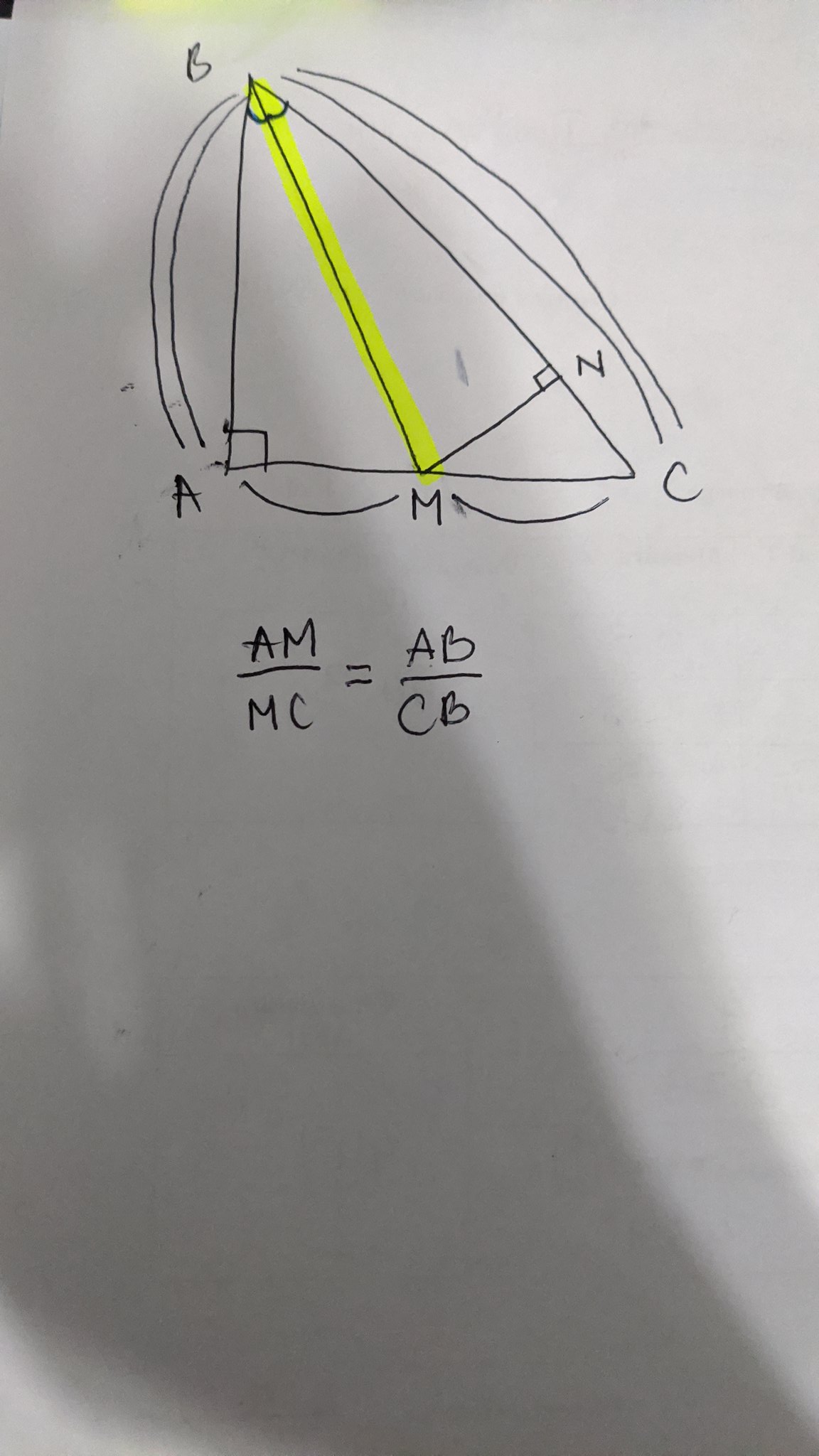The image depicts a meticulously cropped rectangular section of white copier paper containing a mathematical diagram and equation. At the top center of the paper, there is a right triangle labeled with vertices: A at the bottom-left, B at the top, and C at the bottom-right. The right angle is at vertex A and is marked with a small square. A line segment extends from vertex B to the midpoint M of line AC, effectively creating two smaller triangles. Arrows point from A to M, M to C, C to B, and B to A, indicating relationships between these points.

Below the diagram, an essential equation is written:
\[ \frac{AM}{MC} = \frac{AB}{CB} \]

The image also captures the faint shadow of a hand, positioned prominently over the paper, likely belonging to the person who took the picture. This shadow creates a darker silhouette, with a lighter secondary shadow visible behind it.